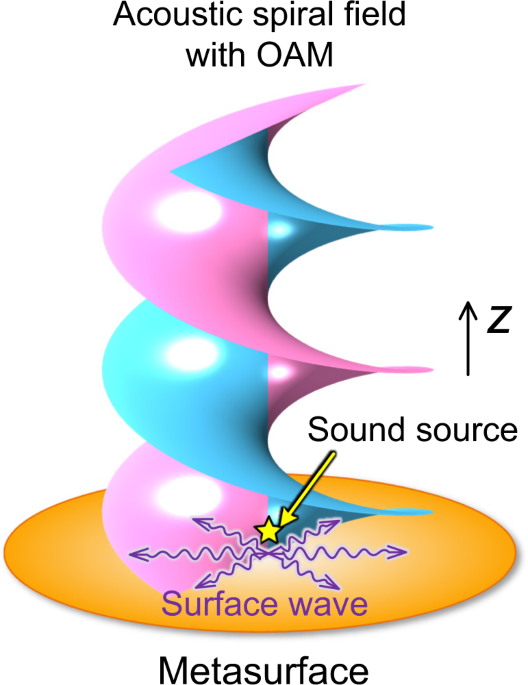The image is an illustrative poster with a plain white background, prominently titled at the top in large black text, "Acoustic Spiral Field with OAM." Central to the image is a spiraling figure rendered in pastel pink and blue hues, twisting in a descending manner along the z-axis, which is indicated by an upward-pointing arrow labeled "Z" on the right side. The spiral, adorned with white highlights, rests atop a foundational yellow oval.

Within the yellow base, there is a central intersection comprised of six crisscrossing wavy purple lines, each terminating with an arrow, reminiscent of a snowflake pattern. Above the convergence point of these lines is a yellow star, highlighted by an upward-pointing yellow arrow labeled "Sound Source." Below these wavy lines, the text "Surface Wave" is detailed in purple.

The base of the yellow oval is marked with the word "Metasurface" in black text. Additionally, a small beam of light bounces off the spiraling form, creating oval highlights on each turn. Despite the detailed depiction of the acoustic structure and elements, the illustration lacks explanatory context for those unfamiliar with the specifics of an acoustic spiral field and its significance.